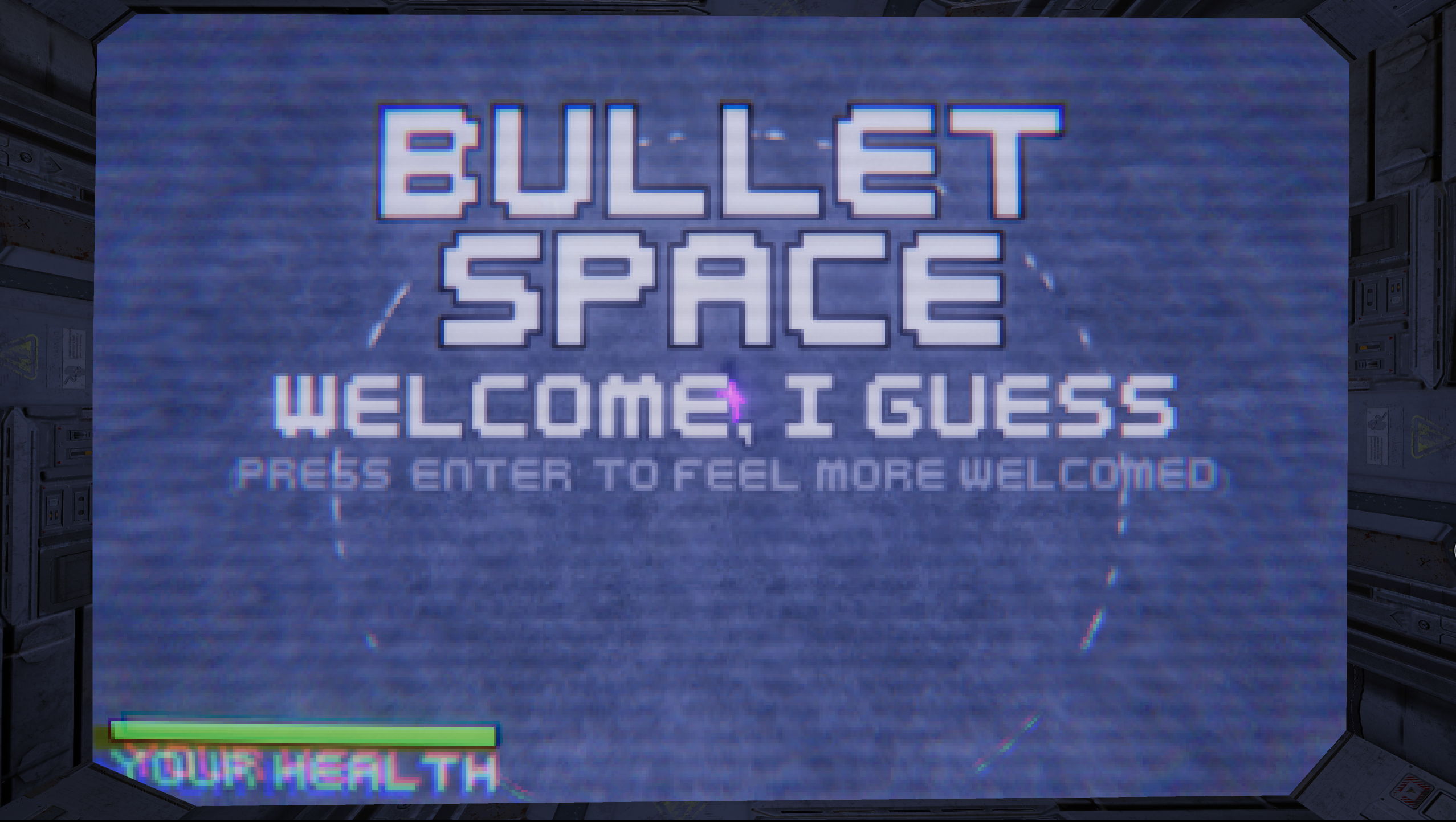The image captures a retro-styled computer game screen with a distinctive feel reminiscent of the 70s or 80s arcade games. The central focus is a blue rectangular background adorned with dark blue and white horizontal stripes, simulating the look of a CRT television. At the top of this blue screen, in large, pixelated, all-caps white letters with a black outline, the text reads "BULLET SPACE" across two lines. Right below, the phrase "WELCOME, I GUESS" appears in a slightly smaller, still pixelated white font. Following this, in a light blue, smaller font, it instructs "PRESS ENTER TO FEEL MORE WELCOMED." In the lower left-hand corner, there is a horizontal green bar, labeled "YOUR HEALTH" in white, capital letters centered beneath it. Surrounding this central blue screen is a dark gray background, which, with its indeterminate details and linear markings, suggests the interior of a spaceship or a similarly enclosed, futuristic environment.